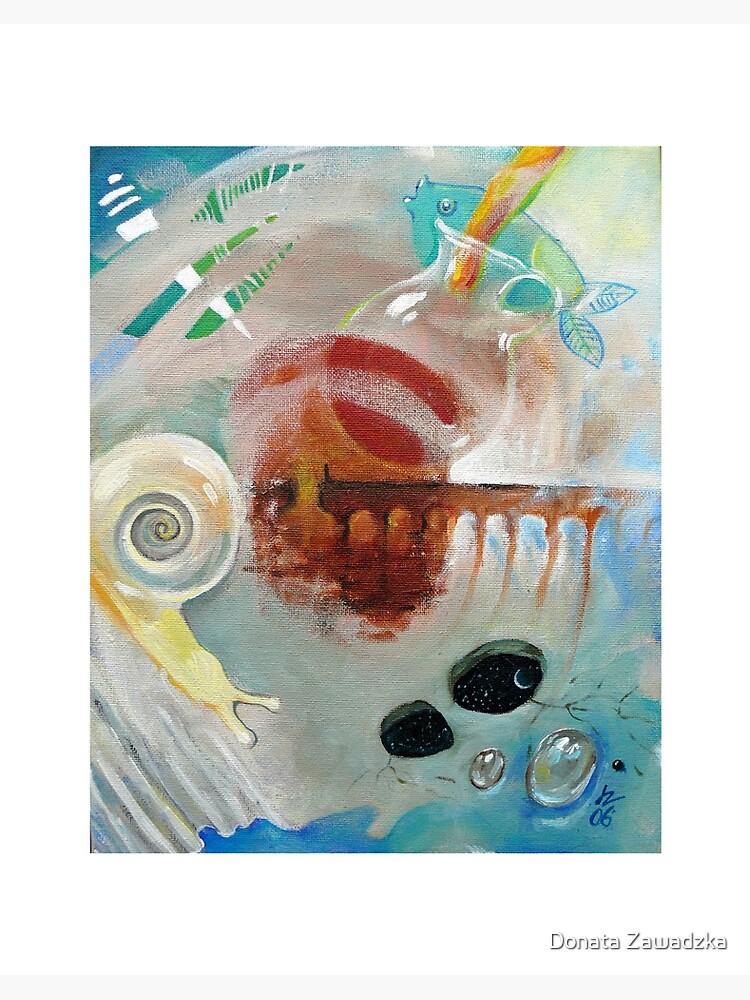This painting on canvas is a vibrant and abstract composition, likely executed in acrylics. The image is dominated by a rich palette of blues and grays, with a variety of sea-themed elements thoughtfully placed throughout. A signature at the bottom reads "Donata Zawadzka," indicating the artist's name.

The artwork is set against a white background with the central focus contained within a vertical rectangle. At the top left, there is a dark blue corner fading into lighter blues. Strikingly, a grey liquid or mist swirls from the bottom left corner across to the top right, adding a sense of fluid motion.

Within this dynamic setting, several key elements stand out. In the upper right corner, a blue fish with an open mouth swims, lending a nautical feel to the piece. Near the center, an ivory, white, and grey snail extends its head downward, curving elegantly towards the center. The snail is juxtaposed with what appears to be an orange and white striped clownfish body, though its head is obscured by a curled human hand, fingers inward around a central comb-like object. Below this, two black scallop shells rest near a cluster of translucent, pearl-like elements that suggest a resemblance to white sea forms or pearls, all set against an undulating blue wave pattern.

This detailed and intriguing composition blends marine life with human elements, evoking both confusion and curiosity, inviting viewers to delve into the depths of its abstract imagery.